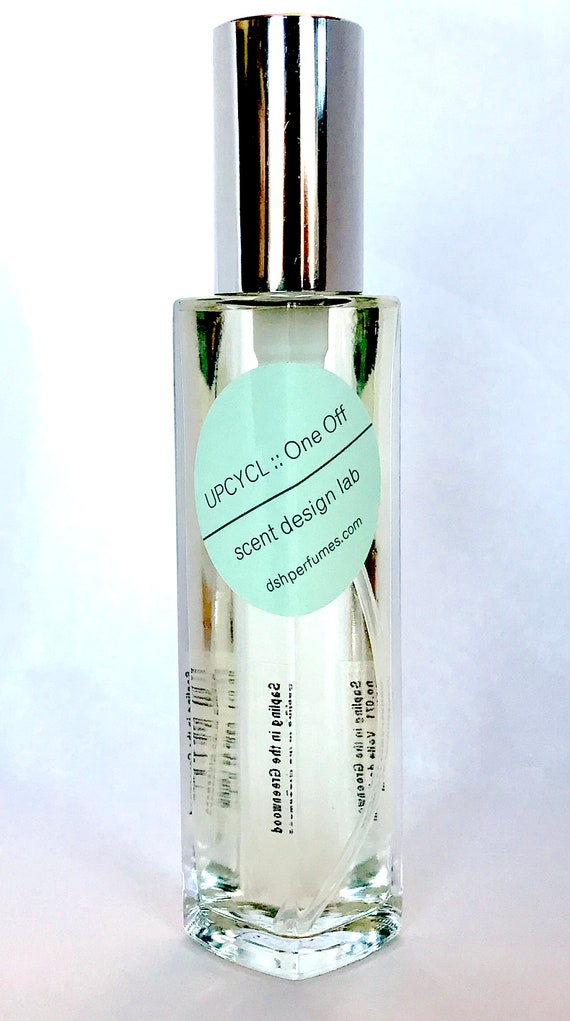This professionally staged, full-color photograph features a vertically rectangular, clear glass perfume bottle with a silver screw-off lid, positioned against a swirling, pastel background that transitions from purplish hues at the bottom to blue and white shades on the sides. The focal point of the image is the bottle's blue, round label, which prominently displays the text "UPCYCL One Off Scent Design Lab" and the website "DSHPerfumes.com." The perfume bottle boasts a cylindrical design with a faceted base, and additional black text is visible near the lower portion of the bottle, though it remains illegible. The photograph, taken with artificial light, exemplifies photographic representationalism realism in product photography.